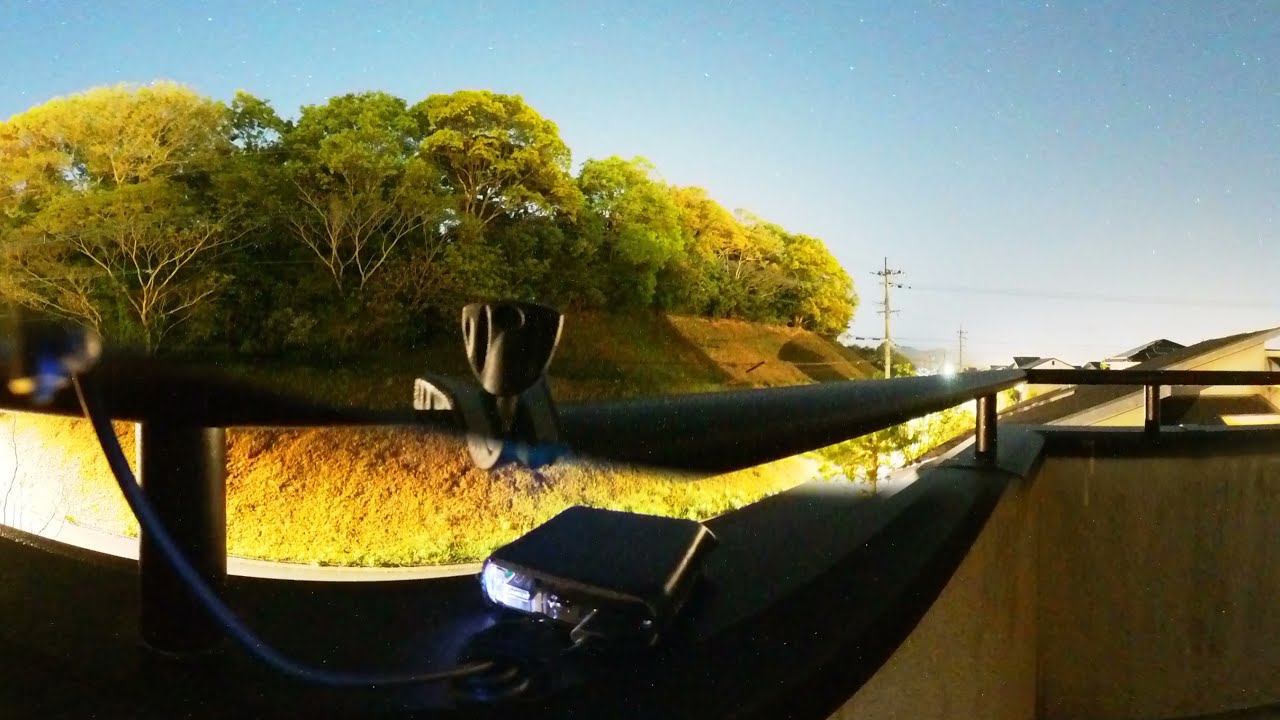This photograph, seemingly taken from the balcony of an apartment building, captures a serene outdoor scene. The image features a black railing that encircles a concrete ledge, suggesting an elevated viewpoint. To the left and prominently in the center, there are lush, green trees with some branches appearing white or brown. The backdrop of the trees is a light blue sky, gradually transitioning into an evening ambiance with faint stars starting to appear, hinting at twilight. Below the trees, there is a small hill blanketed in vivid green grass. Beneath the hill and towards the right, rooftops of tan houses are visible, along with brown telephone poles and various power lines. In the foreground on the balcony, there is a black device with a charging cord attached, adding a touch of modernity to the otherwise natural scene. The soil at the base of the trees appears unusually bright yellow, likely due to a photographic filter. The entire setting gives a tranquil, slightly surreal depiction of a residential neighborhood.